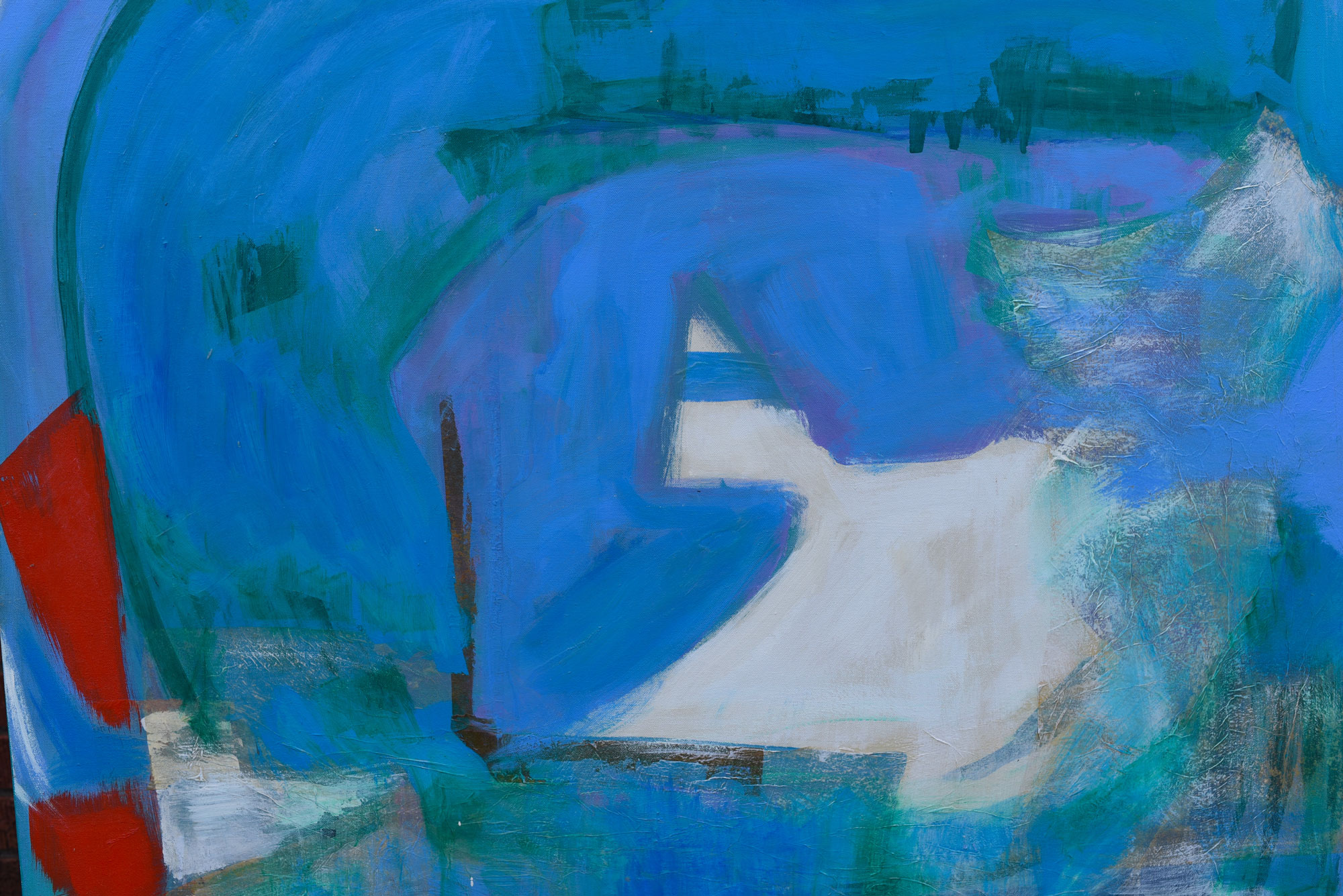This abstract painting features a horizontally oriented composition dominated by varying shades of blue, creating a somewhat shapeless backdrop. The central blue area includes darker smudges and some green patches and lines, which form rounded shapes mostly on the left and top areas of the image. Notably, a white patch resembling a bird's silhouette appears in the middle, with another smaller white shape positioned to the left, accompanied by a pair of red blobs, giving it a superhero-like quality with the semblance of eyes. The upper section of the painting contains a grayish band that has been described as almost street-like. At the bottom left, distinct red splotches, including a triangular shape with curved corners, stand out. Additional smears of white, green, and potentially brown or black paint add to the complexity, with a faint red patch blending into the blue, creating a subtle purple hue. The overall impression is that of viewing a smaller segment of a larger, incomplete image.